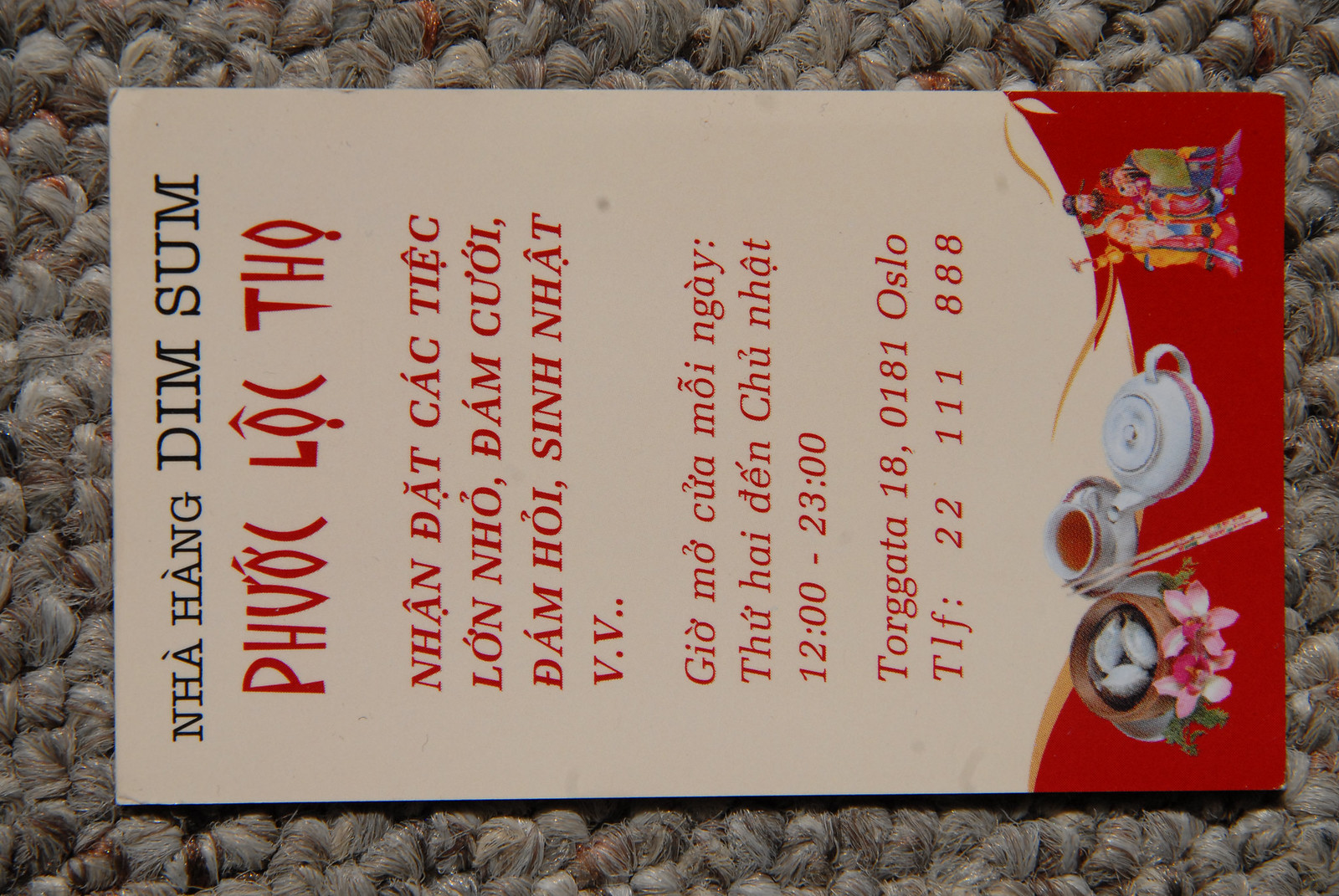This photograph features a book-sized pamphlet placed sideways on a surface that appears to be a tightly woven grey wool material, possibly a rug or a welcome mat. The pamphlet is oriented horizontally but meant to be read vertically. The background surface gives a textured, cozy impression with its woolen look.

The pamphlet is primarily in Vietnamese, with black and red text. The prominent black text at the top reads "Nga Hang Dim Sum." Below this, in stylized red letters, it states "Phuoc Loc Tho." Further down, there's a paragraph in red capital letters: "Nam Dat Khac Tiec Lan Ngo Dam Huey Dam Huey Sinh Nhat," followed by "V.V..". Another section includes operating hours in Vietnamese, "Gio Mo Cua Moi Ngay Tu Hai Den Chu Nhat," listed as 1200 to 2300 hours.

At the very bottom of the pamphlet, which is colored in a red wavy strip, there are images of dim sum in a bamboo steam box adorned with flowers, a cup of tea with a teapot, and an illustration of a traditional Chinese emperor in red attire, possibly holding a sword. The pamphlet also includes an address, "Tor Gata 18, 0181 Oslo," and a contact number, "TLF: 22 11 18 88," indicating that it advertises a Vietnamese restaurant located in Oslo, Norway.